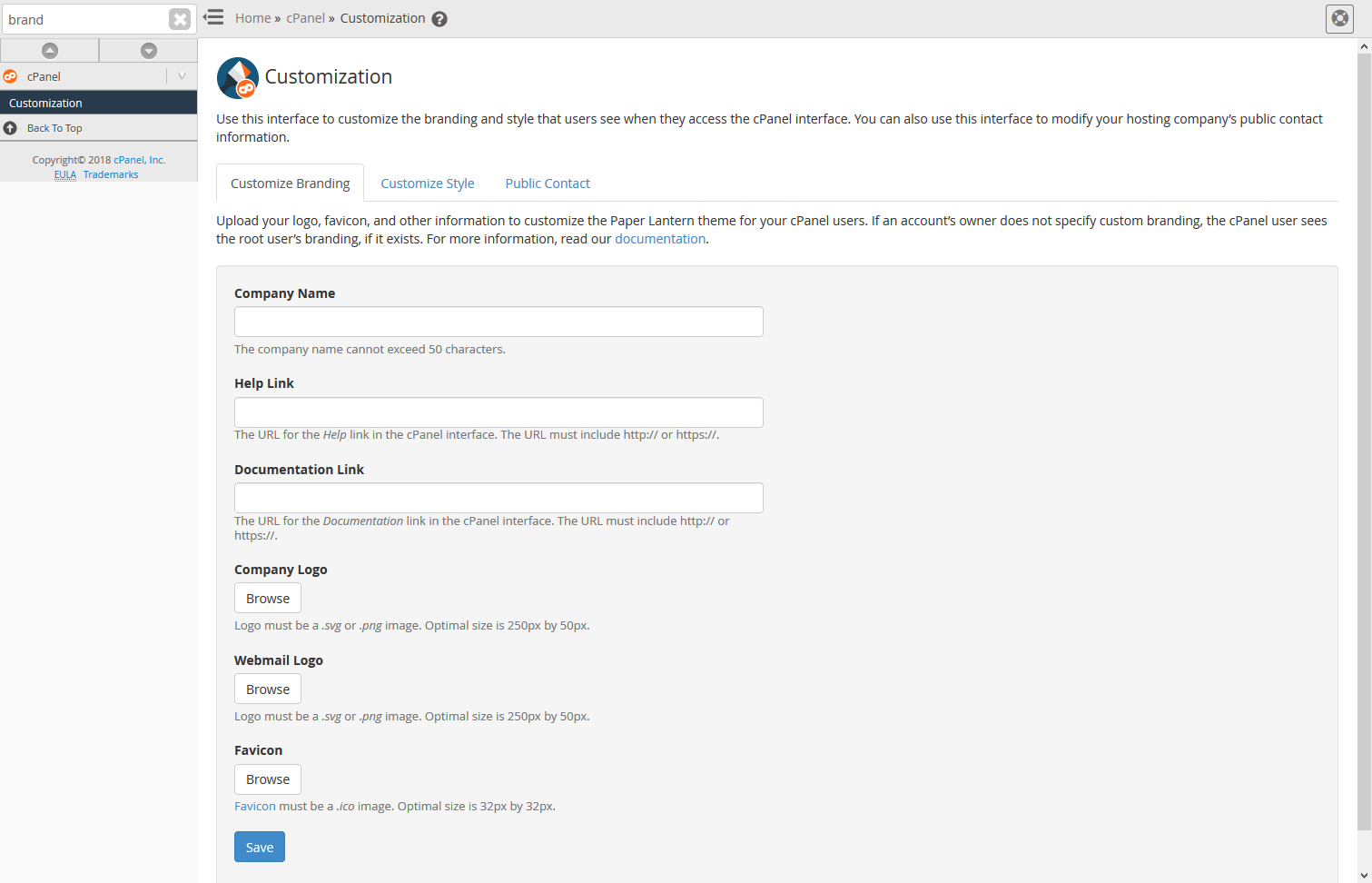The image depicts an interface screen designed for customization of branding and style settings for a channel. At the very bottom of the screen, there is a prominent blue button labeled "Save." At the top of the screen, the word "Customisation" is displayed along with a figure icon or tab. The interface provides options for customizing the channel's branding and aesthetic that users will see when they access it. Additionally, it allows for modifications to the hosting company's public contact information.

In the middle of the interface, several customization options are presented. There is a box designated for entering the company name, which is currently blank, allowing up to 50 characters of input. Beneath this are areas to enter URLs for a help link and a documentation link, respectively. There are also designated fields where the user can upload a company logo, a webmail logo, and a favicon. Each of these fields is designed to allow the insertion of the corresponding items.

On the top right-hand corner of the image, there is an "x" icon that users can click to remove elements from the interface. In the top left-hand corner, there is a search bar where, in this instance, the term "brand" has been entered. Situated beneath the search bar are two directional arrows. Below these arrows are boxes labeled "Channel" and "Customisation," followed by another box labeled "Back to the Top."